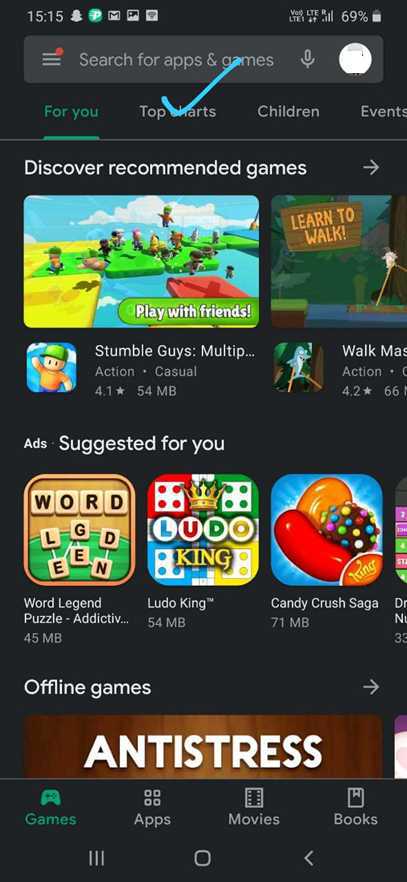This blurred and somewhat pixelated image captures the screen of a handheld device. In the upper-left corner of the screen, the time is displayed as "15:15" alongside a Snapchat icon and several other icons, which include an email icon and a picture icon. The top-right corner reveals network information that reads "Void LTE," accompanied by a Wi-Fi icon, a battery percentage at 69%, and a battery icon. 

Centrally located on the screen is a search bar. On its left side, there is a "More" icon, and the middle of the search bar prompts users with the text "Search for apps and games." To the right of this prompt is a microphone icon. 

Below the search bar, four tabs are visible, labeled from left to right: "For You," "Top Charts" (highlighted with a blue checkmark), "Children," and "Events." Beneath these tabs, more text is partially visible.